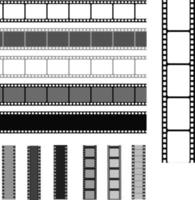The image features a series of cartoonish film strips against a white background, predominantly rendered in black, white, and varying shades of gray. On the left side, five identical film strips are arranged horizontally in a top-to-bottom sequence, with each stripe distinctively colored: the top strip is in black and white, followed by a strip in white and gray, the next in light gray and white, then black and gray, and the final one in solid black. To the right, a close-up of the top black-and-white film strip is positioned vertically. At the bottom of the image, six smaller film strips, repeating the same coloration patterns, are aligned vertically side-by-side with white spaces between them. Each film strip consists of rectangular cells, some with dividing bars and others without, reflecting various levels of opacity and shades.